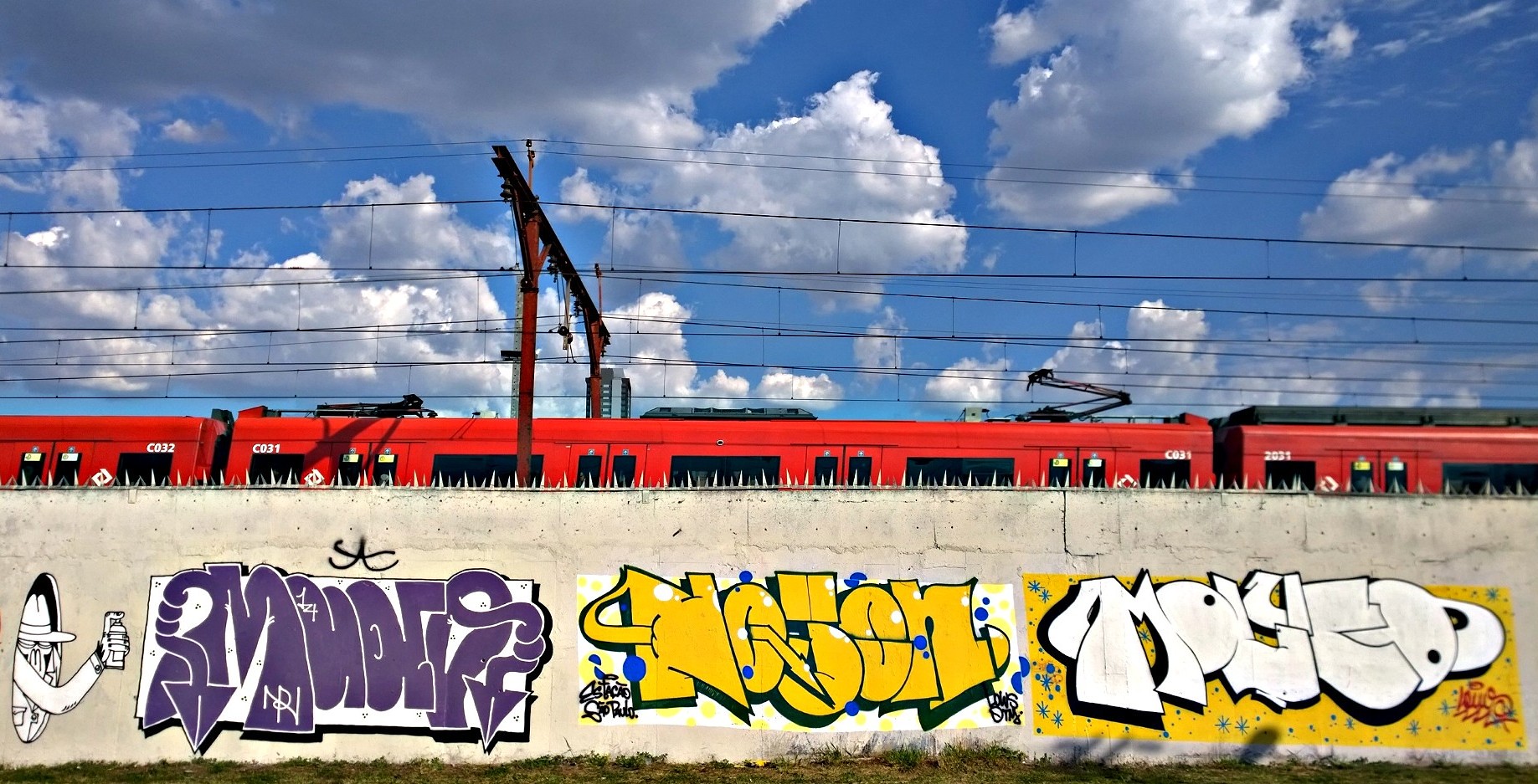In the image, a vibrant red trolley train, reminiscent of Chicago's elevated loop, is partially visible, its defining serial numbers CO32, CO31, and 2031 marking each car. The train navigates along its elevated track, intersected by a web of power lines that blend into a sky filled with big, white clouds against a brilliant blue backdrop. Below the train is a stark white wall topped with silver spikes, adorned with a variety of graffiti. Prominently, the wall features an illustration of a sneaky looking character wearing a trench coat and hat. Surrounding this character are multiple graffiti tags in vivid colors: purple and white, yellow on a white background, white on yellow, and a striking red and black signature. The image is set outdoors and is well-lit, capturing the energy and artistic expressions of urban life.